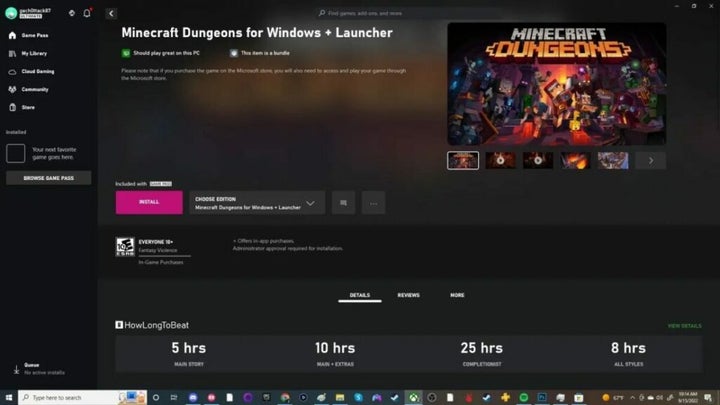This screenshot showcases the Minecraft Dungeons application page on an online platform. Dominating the center of the screen is a large black box with various interactive elements. On the left side, there are multiple tabs for navigating through the menu options. 

At the top of the interface, there is a circular icon, and to its right, a bell icon marked with a red notification dot. Moving into the black box's main content, the screen displays the text "Minecraft Dungeons for Windows + Launcher."

Below this heading, a prominent pink banner labeled "Install" indicates the process to download and install the game onto a computer. Adjacent to the "Install" banner, there is an option labeled "Choose Edition" with a drop-down arrow for further selection. Next to this, a small square icon featuring a message symbol appears, followed by another dark square icon with three ellipsis points, suggesting more options.

Additionally, the screen includes an image from Minecraft Dungeons, representing the popular computer game. Beneath this image are multiple thumbnail squares, likely linked to various videos that preview different aspects of gameplay. These video links provide examples of the in-game experience, offering a visual guide to potential players.